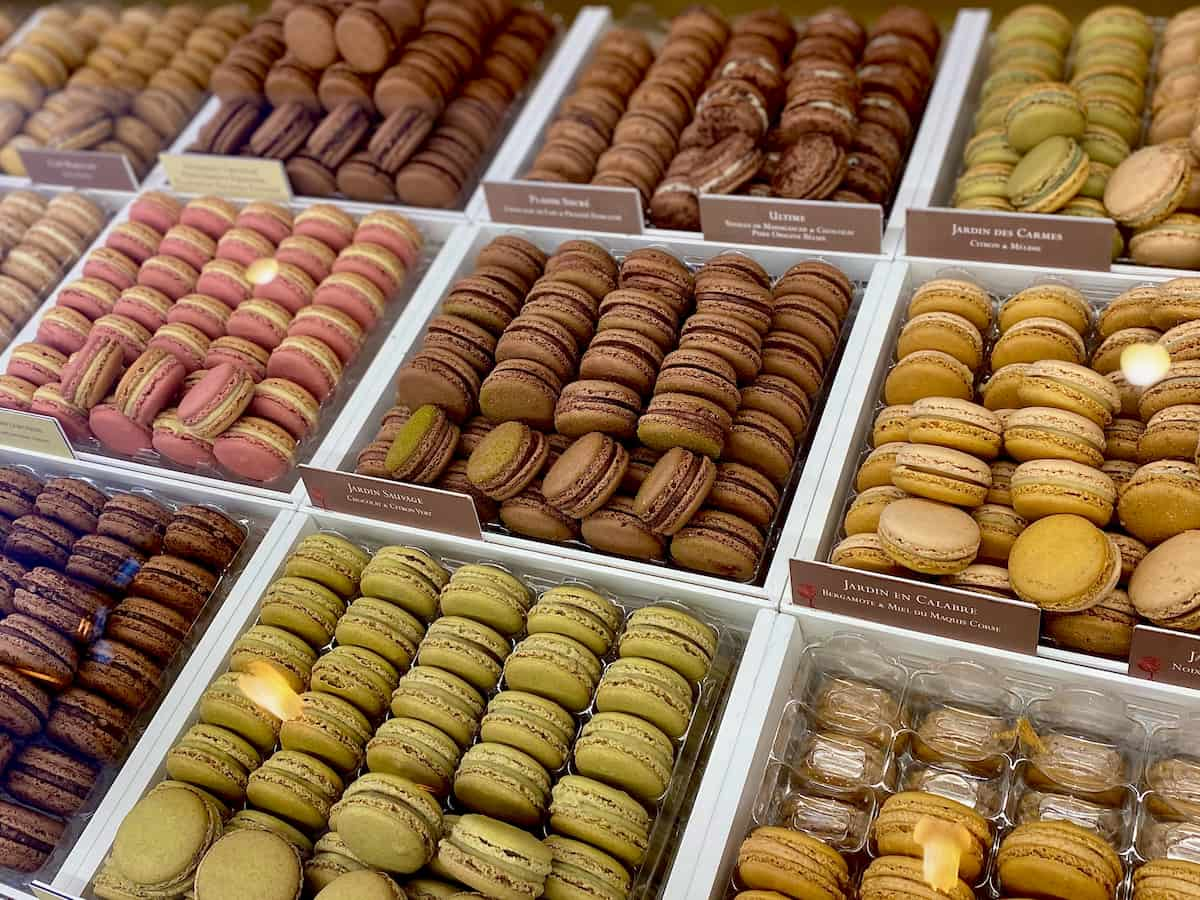The image depicts an assortment of cookies displayed in a shop, possibly a bakery or a grocery store. The cookies are arranged in neatly separated white compartments, creating a visually appealing layout. Starting from the bottom right corner, there are light brown cookies, partially covered by transparent plastic. Directly behind these, more cookies are visible. Moving to the left, there are intriguing green cookies with a creamy filling, resembling small sandwiches or hamburgers. These green cookies, along with the others, have a brown label between sections with unreadable white text.

Centrally, a cluster of dark brown cookies can be seen, with some exhibiting a greenish tint. Towards the left side and middle, there are cookies with pink tops and yellow bottoms. At the very bottom left, there are extremely dark brown cookies, especially noticeable around the cream-filled center. The top rows feature light brown cookies to the top left, green cookies to the top right, dark brown ones towards the top, and pink cookies in the mid-left. There's also the presence of beige cookies at the right and yellow-hued cookies at the bottom right. The entire display appears meticulously organized in a grid of square containers, portraying a vibrant variety of flavors and colors.